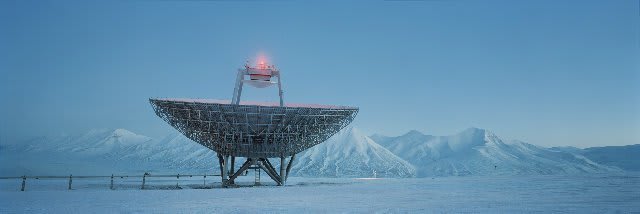The image captures a panoramic winter landscape dominated by hues of blue. The upper half of the scene is filled with a clear, blue sky that meets a uniform mountain range extending across the width of the image. These mountains are modest in height, cloaked in shades of blue and dusted with white snow. In the foreground, the ground is covered in a pristine layer of snow. To the left, a slender fence composed of black posts and a single line runs partially into the frame. Near the center, slightly offset to the right, stands a large, scientific structure that resembles a parabolic dish. This dish, mounted on triangular legs, is dark gray and oriented upwards as though it is collecting data from the sky. A distinctive feature of this apparatus is an extension rising from the center of the dish, crowned with a pinkish-red light, possibly indicating its active status in data collection. The image conveys a sense of serene, cold stillness juxtaposed with the technological presence amidst nature.